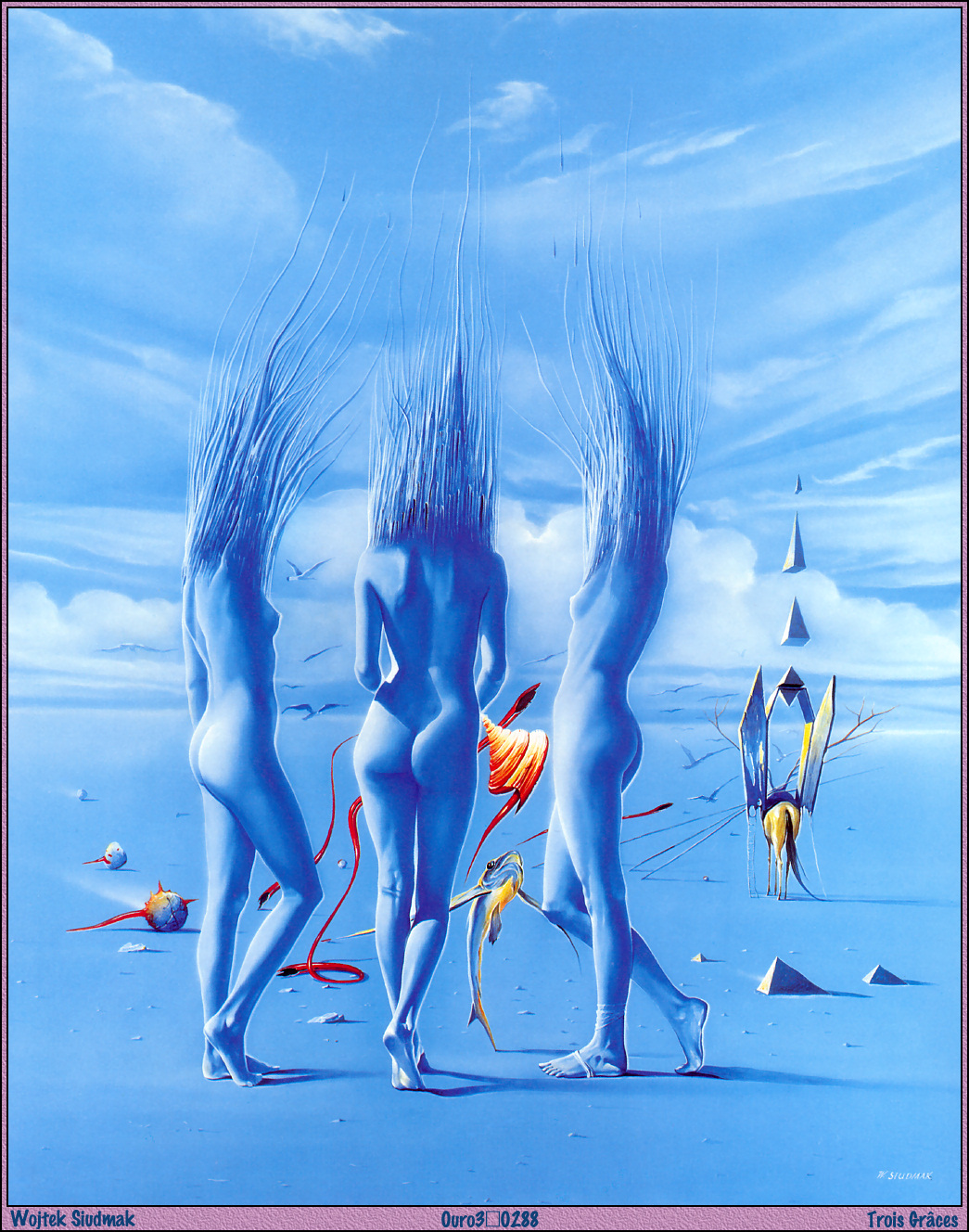The artwork is a surreal, digital creation predominantly rendered in blue tones, ranging from light to dark, but not extremely dark, creating a cohesive blue palette. The composition features a trio of abstract, feminine forms standing in the foreground, their heads replaced with intricate, tree-root-like structures or blue grass. The bodies of these figures are entwined with medium-toned colors that blend seamlessly between the background and the foreground.

The scene is set against a backdrop of blue-tinted clouds, enhancing the ethereal quality of the piece. Below the figures, the ground also maintains this blue motif, although it mimics the sandy texture. Various fantastical elements inhabit the scene including an orange and red conch shell centrally positioned, a yellow and blue fish balanced delicately on the tip of a flipper, and an antelope-like creature facing away on the right-hand side. Additionally, two ball-like creatures with reddish hues and swirling snake-like ribbons add to the surrealism.

Text details feature prominently at the bottom of the image: the artist’s name, "Wojtek Siudmak," is inscribed, as well as the title "Trois Grâces." There is also an enigmatic code, "OURO30288."

This fusion of elements melds the fantastical with the abstract, invoking a sense of otherworldly wonder.